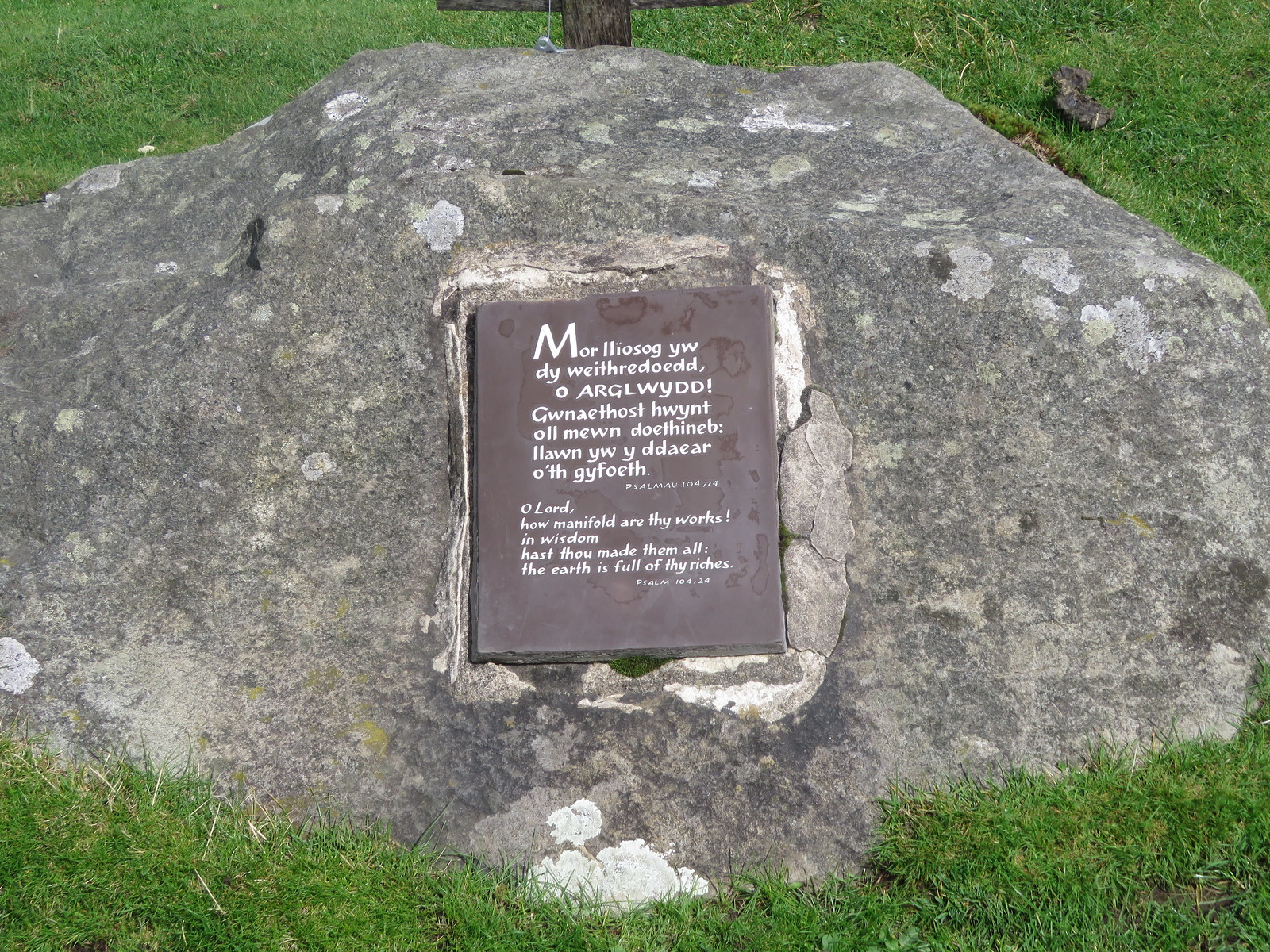The image features a large, dark gray rock situated on a bed of green grass, with a portion of a cross visible behind it. Embedded in the center of the rock is a rectangular metal plaque that bears white engraved letters. The plaque's upper paragraph is written in a foreign language, while the bottom section, in English, reads: "O Lord, how manifold are thy works; in wisdom hast thou made them all: the earth is full of thy riches." Surrounding the text are traces of wear, with small splashes of lighter colors possibly from other rocks or damage. Below the passage, there is additional smaller white text that is too small to discern. The rock appears weathered, contributing to the sense of reverence and history encapsulated by the scene.